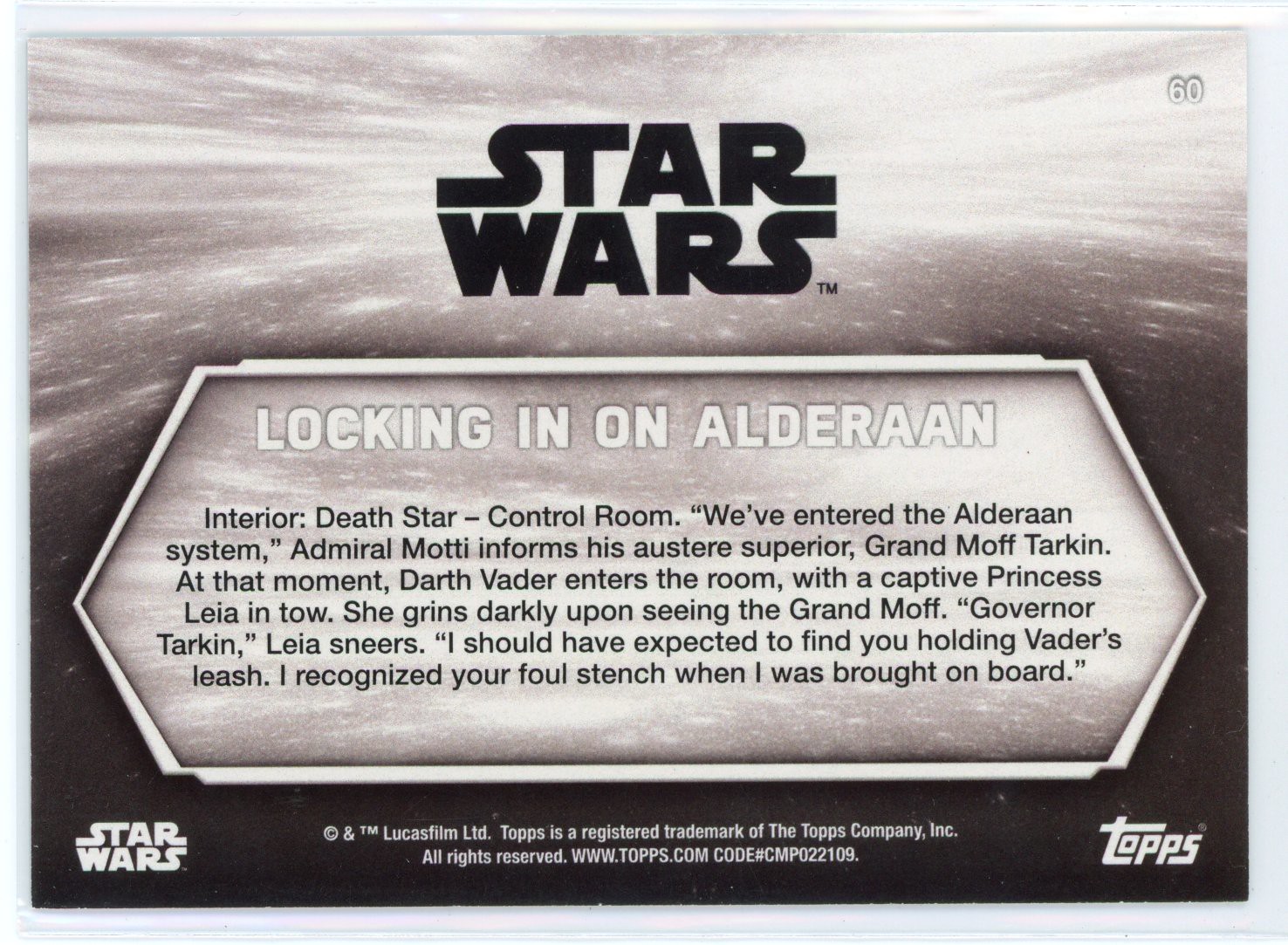This image is a detailed grayscale trading card featuring a Star Wars scene and associated details. The background transitions from a grayish white, reminiscent of a cloudy or starry sky, down to black. The upper portion of the image prominently displays the Star Wars logo in bold black letters, and to the right, the number 60 is printed in white. Below this, a white trapezoidal frame outlines the main text area, which shares the background's light gray and white tones.

Inside the trapezoid, large white letters spell out "Locking in on Alderaan." Beneath this, in smaller black text, it reads, "Interior, Death Star, Control Room. 'We've entered Alderaan system,' Admiral Madi informs his austere superior, Grand Moff Tarkin. At that moment, Darth Vader enters the room with a captive Princess Leia in tow. She grins darkly upon seeing the Grand Moff. 'Governor Tarkin,' Leia sneers. 'I should have expected to find you holding Vader's leash. I recognized your foul stench when I was brought on board.'"

At the bottom of the card, the left corner features the Star Wars logo in white, followed by the Lucasfilm and Topps copyrights. Conversely, the bottom right corner displays the white Topps logo. The card's overall theme is designed to evoke a sense of motion through space, with the upper background resembling a blurry, fast-moving starry sky. The dense text and iconic logos suggest the card is part of an advertisement or collectible series related to the Star Wars franchise.